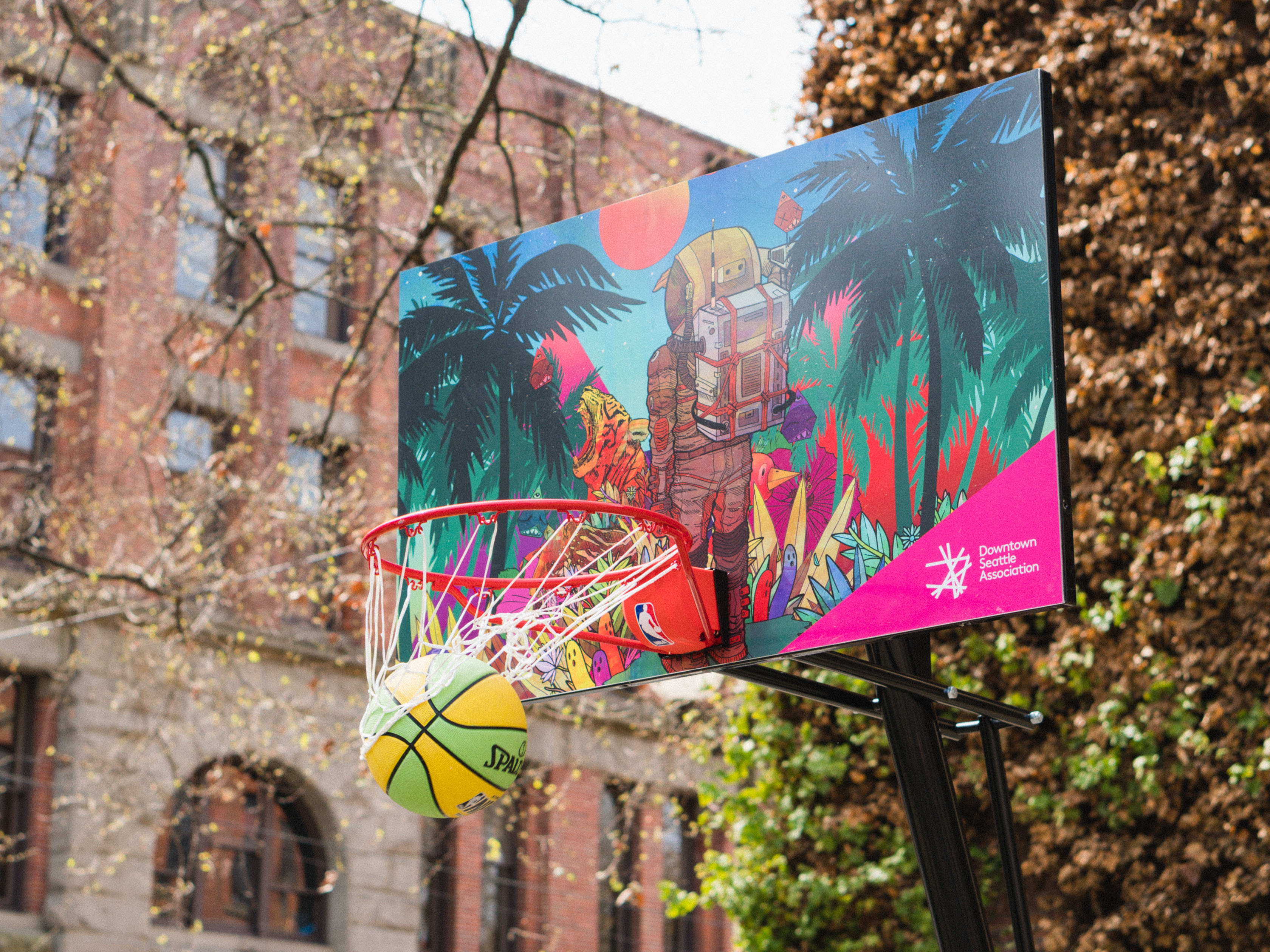This photograph captures an outdoor basketball hoop framed against a detailed and colorful backdrop. Centered in the imagery is a vibrant basketball backboard adorned with a highly artistic and vivid graphic. The backboard showcases an astronaut-like figure in brown and red gear, complete with a backpack, navigating a jungle scene that includes two palm trees, a distant planet, and a tiger at the bottom right. This corner also features a pink triangle banner that reads "Downtown Seattle Association." 

The rim of the hoop is classic orange, with a white net that is currently funneling a Spalding basketball downwards. This basketball stands out with its unique alternating green and yellow panels. The hoop is mounted on a black tubular steel frame, which partially obscures the visibility of the court itself. 

Background elements add to the complexity; on the left, a large red and brown brick and stone building with several arched windows—an imposing three to four stories high—provides a textured backdrop. To the right, there is lush foliage, including a brown bush with sprouting green leaves and a tree branch adorned with small yellow leaves. Additionally, vines crawl up a wall in the background, blending green and gold hues to complement the scene. The overall composition creates a dynamic interplay between urban art and natural elements, emphasizing the juxtaposition of structure and nature.